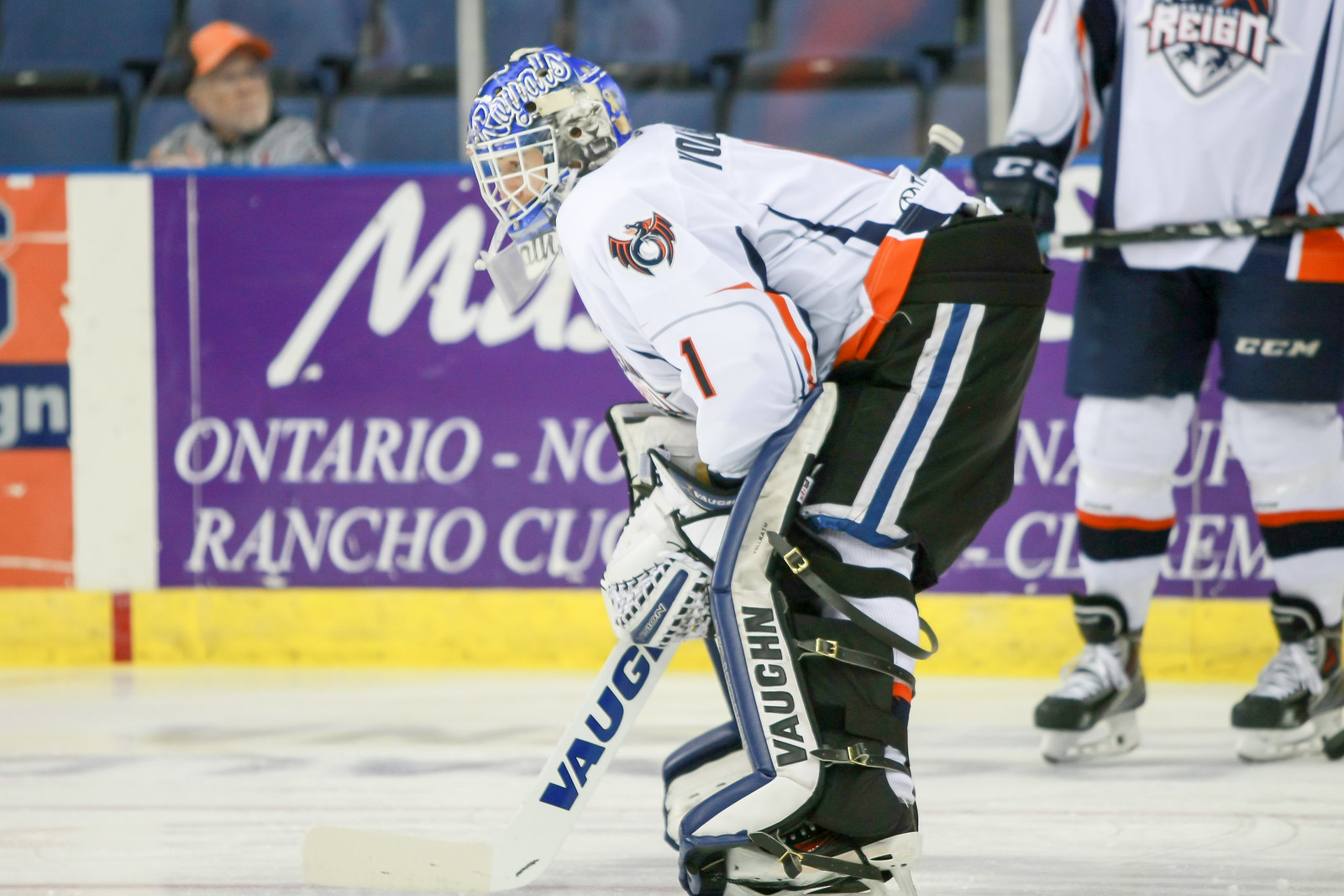The photograph captures an intense moment on an ice hockey rink featuring two hockey players in full gear. The central figure, viewed from the side profile, is bent over at the waist, focused intently on a puck. This player wears a white jersey with orange, blue, and yellow accents, black pants with a white and blue stripe, and a blue helmet emblazoned with "Royals." Their padded goalie gear, including large gloves and leg pads, is clearly visible. To the right of this player stands another teammate, visible from the chest down, wearing a similar uniform with a "Rain" emblem on the jersey. Both players are equipped with hockey sticks, poised on the white ice rink. In the background, a crowd is discernible, seated in blue bleacher chairs behind a protective plastic wall. Prominently displayed is an advertisement sign with a purple background and white text, reading "Ontario Rancho." Among the spectators, a man sporting an orange baseball cap can be spotted. The image captures the dynamic energy and anticipation typical of an ice hockey game in a stadium setting.